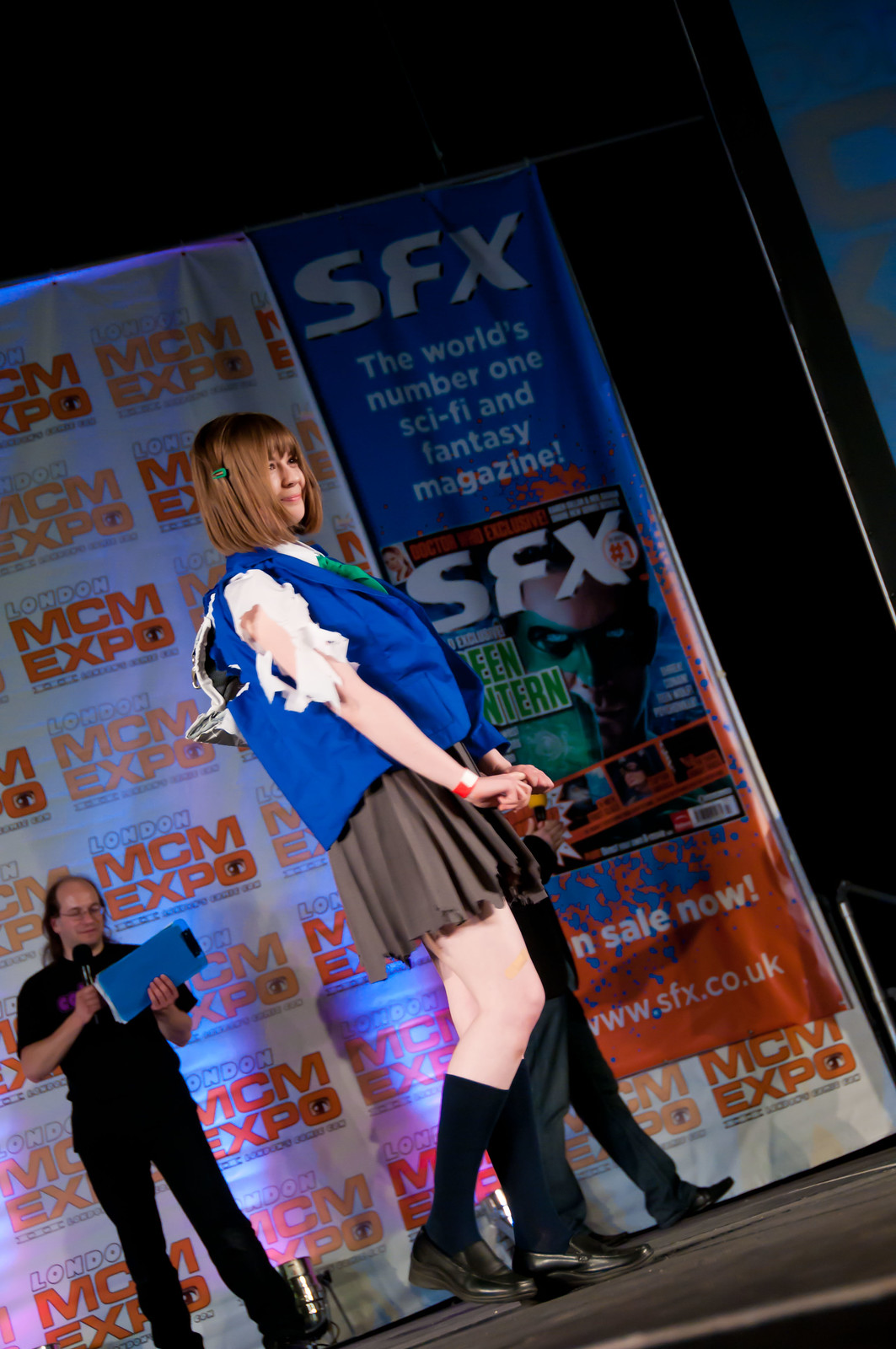This photograph captures a dynamic moment on a tilted indoor stage, angled about 30 degrees counterclockwise. At the forefront, a smiling Asian girl with brown hair is in side view, dressed in a blue vest, a brown pleated miniskirt, black knee-high socks, and brown loafers. Behind her, two more people are present on the stage; one is fully visible, the other partially. Notably, one person holds a microphone and blue clipboard, seemingly an announcer. He is balding with long hair at the back and wears a black outfit. The backdrop features a large, text-filled poster with "SFX, the world's number one sci-fi and fantasy magazine" prominently displayed, along with the "MCM Expo" title and various logos and advertisements in three vertical columns.